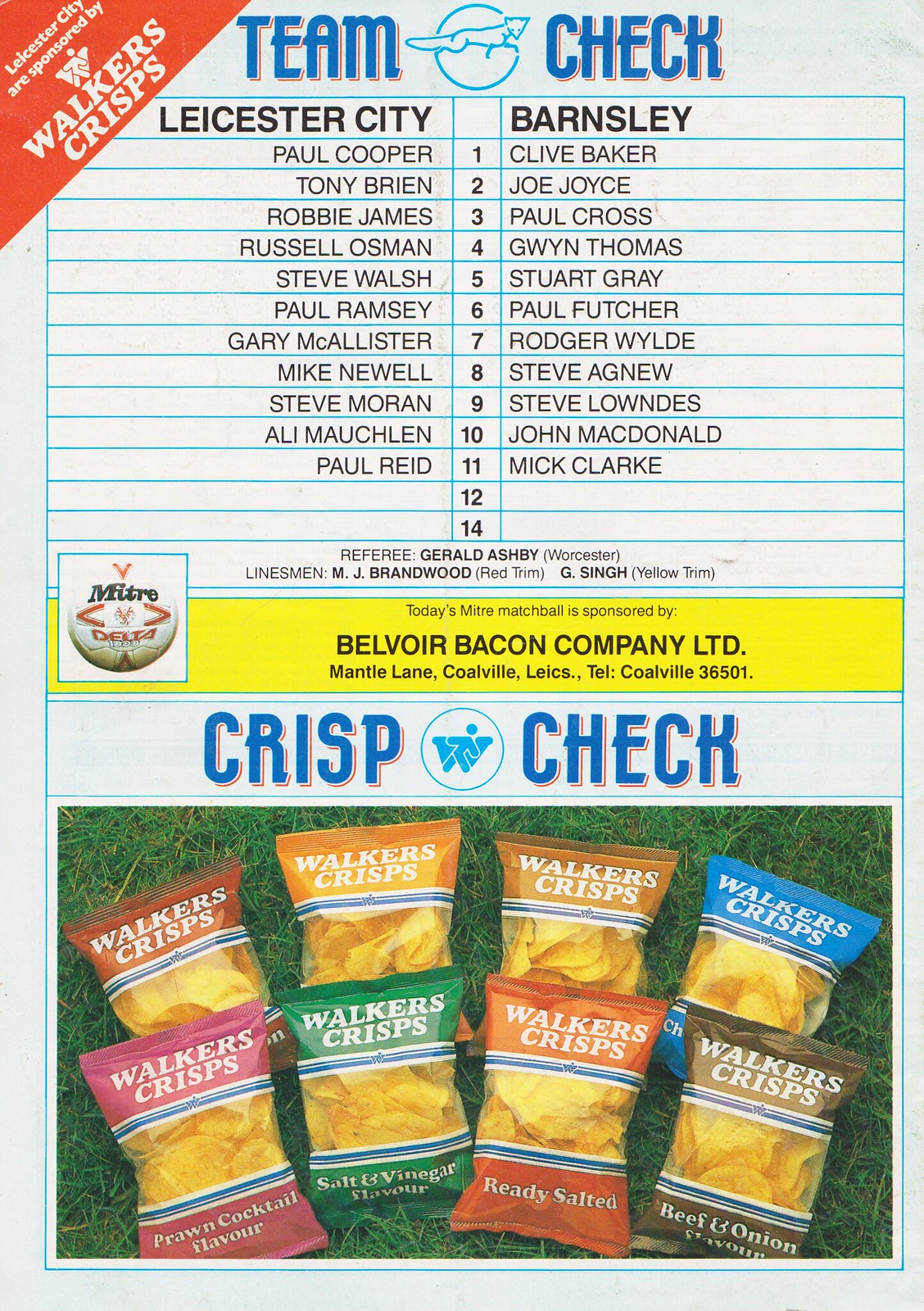This image is the cover of a program or flyer for a soccer game, likely between Leicester City and Barnsley. The top half has a white background with blue lines, resembling loose leaf paper. The title "Team Check" is prominently displayed in blue at the top, with a teal circle logo featuring a fox peeking out. In the upper left corner, there's a red notch with white text stating that Leicester City is sponsored by Walker's Crisps. Below the title, a table lists the rosters of both teams: Leicester City on the left and Barnsley on the right, with positions numbered from 1 to 14.

In the middle section, a yellow banner with black text announces, "Today's Mitre Match Ball is sponsored by Belvoir Bacon Company, LTD," including the company's address and phone number. At the very bottom of the page, the section labeled "Crisp Check" displays eight different flavors of Walker's Crisps on a grass background, including prawn cocktail, salt and vinegar, ready salted, and beef and onion.